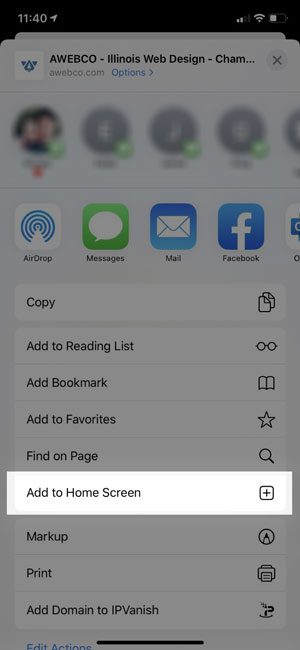The image showcases the user interface of Webco Illinois, a web design application. The top of the screen displays the current time, 11:40, alongside indicators for battery life and Wi-Fi connectivity. The main interface features several options: 'Airdrop' for wireless file sharing, 'Messages' for text communications, 'Email,' 'Facebook,' 'Copy,' 'Add to Reading List,' 'Bookmark,' 'Add to Favorites,' which is indicated by a star icon, 'Print,' and 'Add Domain to IPVanish,' a VPN service.

Highlighted prominently in white, possibly due to user selection, is the 'Favorites' option featuring a star icon. Also visible is an open book icon, likely representing the 'Reading List.' The 'Magnifying Glass' icon, used for search functions, is distinctly bright, making it stand out from the other icons. This detailed user interface provides a comprehensive array of tools for robust web management and design.